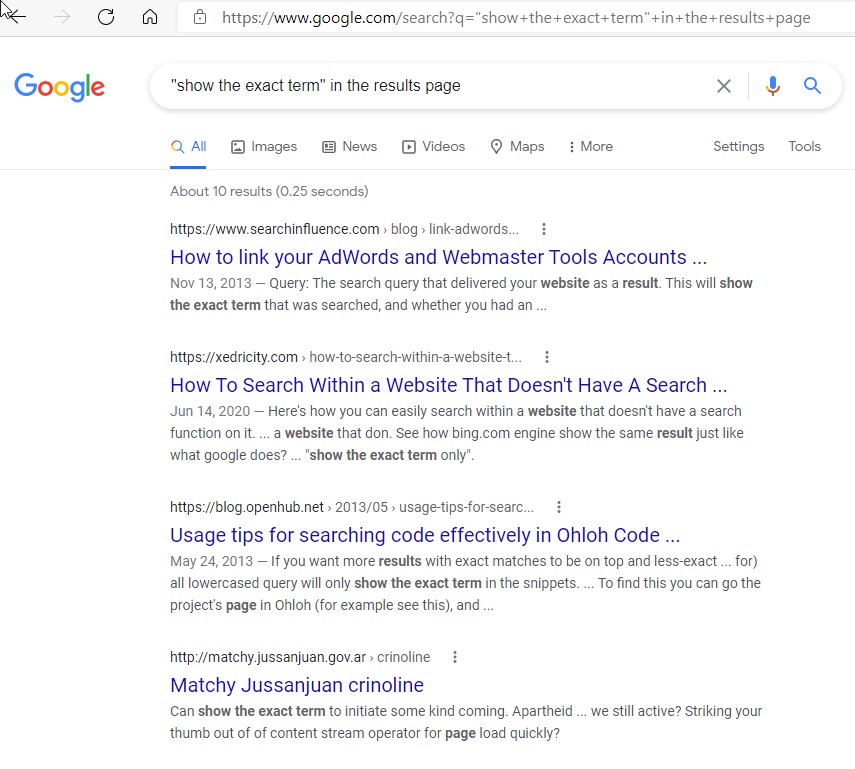The image depicts a Google search results page. The search query, "show the exact term in quotations in the results page," is prominently displayed. The search engine returns approximately 10 results in 0.25 seconds. The top URL in the browser's address bar reads: `https://www.google.com/?q="show+the+exact+term+in+quotations+in+the+results+page"`.

The visible search results include:
1. A guide on linking AdWords and Webmaster Tools accounts.
2. Instructions on how to search within a website that lacks a search feature.
3. Tips for effectively searching code within OLO code.
4. Results from Matchly, Just and Juan, and Crinoline.

At the top of the browser, several navigation and utility buttons are visible: a home button, a refresh button, a grayed-out forward arrow, a black back arrow, and a white mouse cursor positioned on the screen. Additionally, various Google search tabs such as "All," "Images," "News," "Videos," "Maps," "More," "Settings," and "Tools" are accessible just below the search bar.